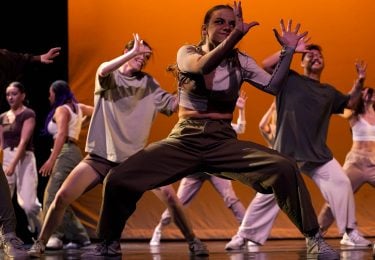The image is a landscape-oriented color photograph depicting a dynamic scene of a dance performance on a stage. Dominating the background is a bright orange curtain that spans across the majority of the image, with a black panel occupying about one-fifth of the width on the far left where the curtain ends. In the foreground, a man in a costume is prominently featured, crouched down with his legs spread wide and his hands raised in the air, performing a vigorous dance move. Behind him, two more dancers mirror his stance, and further back, another row of dancers also adopt the same power pose, all facing the top right section of the image. The performers are diverse, representing a mix of races and genders, and are dressed in a variety of clothing styles ranging from pants to shorts, generally favoring baggy attire. On the left side of the stage, some additional dancers are visible, facing away from the primary group and seemingly engaged in conversation or preparation. The overall style of the photograph is realistic and representational, effectively capturing the energy and diversity of the dance performance.